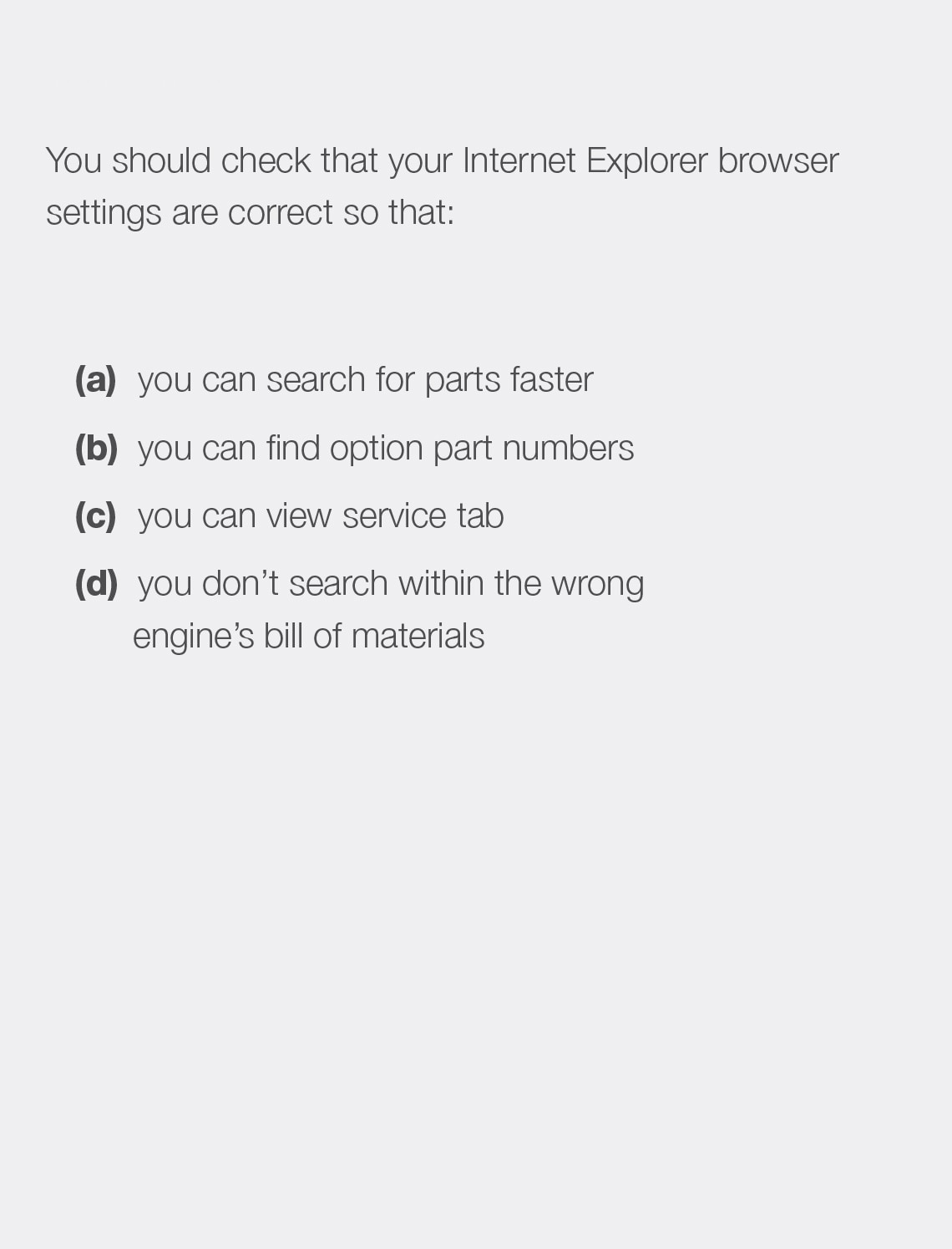The image features a light gray box with a slightly purple hue as the background. At the top of the box, there is a clear directive in light black text instructing users to check their Internet Explorer browser settings. This is emphasized to ensure that users can: (A) search for parts faster, (B) find option parts numbers, (C) view the service tab, and (D) avoid searching within the wrong engine bill of materials. Below this directive, there is a considerable blank space, creating a gap between the sentence at the top and the list of options labeled A, B, C, and D. The letters A, B, C, and D are enclosed in parentheses and are displayed in a bold color to stand out from the rest of the text. The overall minimalistic design of the image leaves much of the space unoccupied.